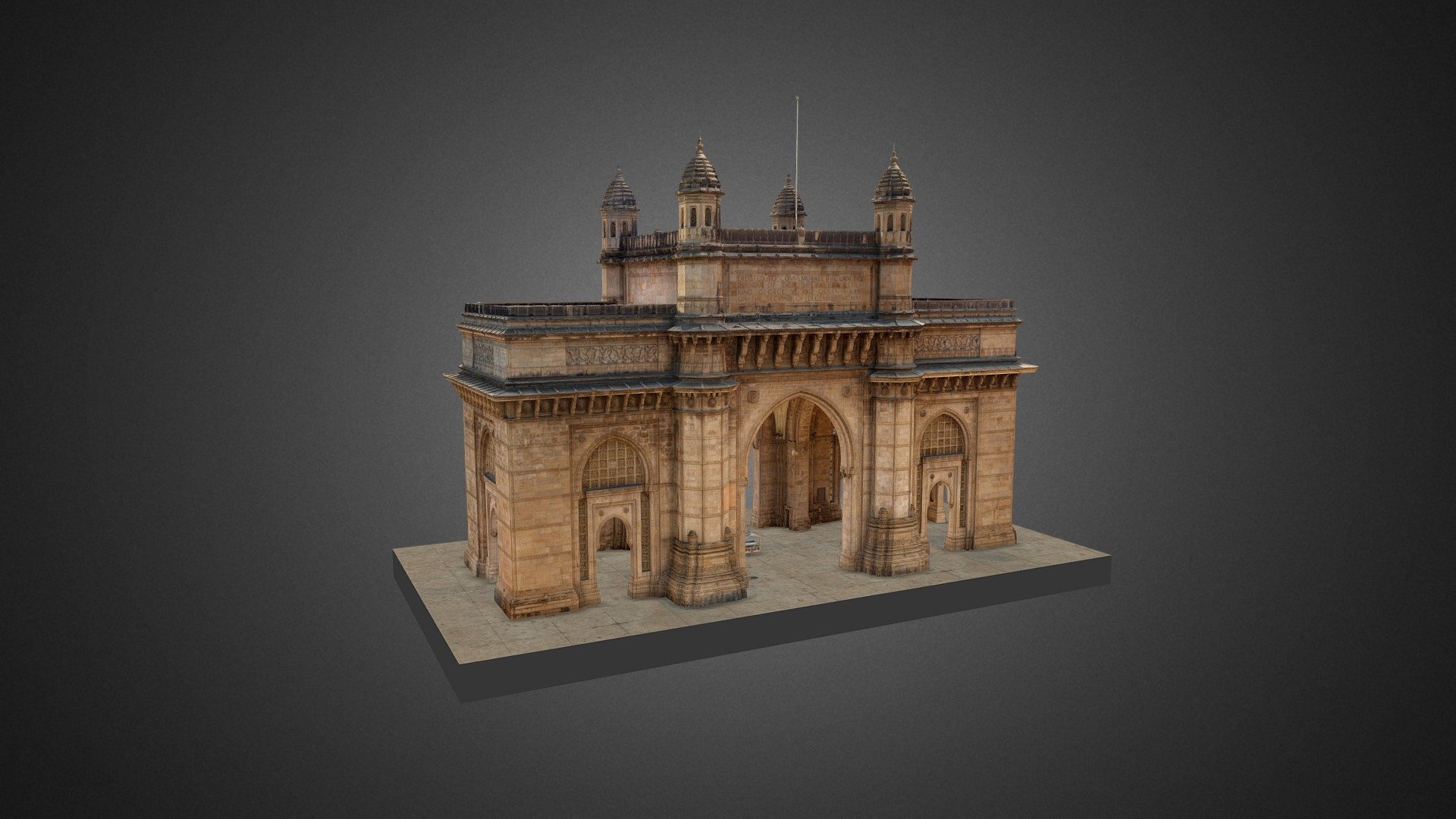This image appears to be a detailed 3D rendering of a medieval-style entranceway set against a dark gray gradient background. The focal point is a large, camel-colored stone structure reminiscent of a historical building. Central to the composition is a prominent, large oval archway that suggests it could accommodate a descending gate, surrounded by two smaller, similarly shaped archways on either side. Each archway is supported by columns, intricately carved with medieval designs. The structure is topped with four pointed towers, two at the front and two at the back, adding to its castle-like appearance. The building rests on a stage-like platform composed of light brown to beige slate tiles. The overall ambiance, combined with the rendering's highly detailed and somewhat realistic finish, evokes the aesthetic of an ancient gate or entryway to a grand, possibly fortified city or palace.